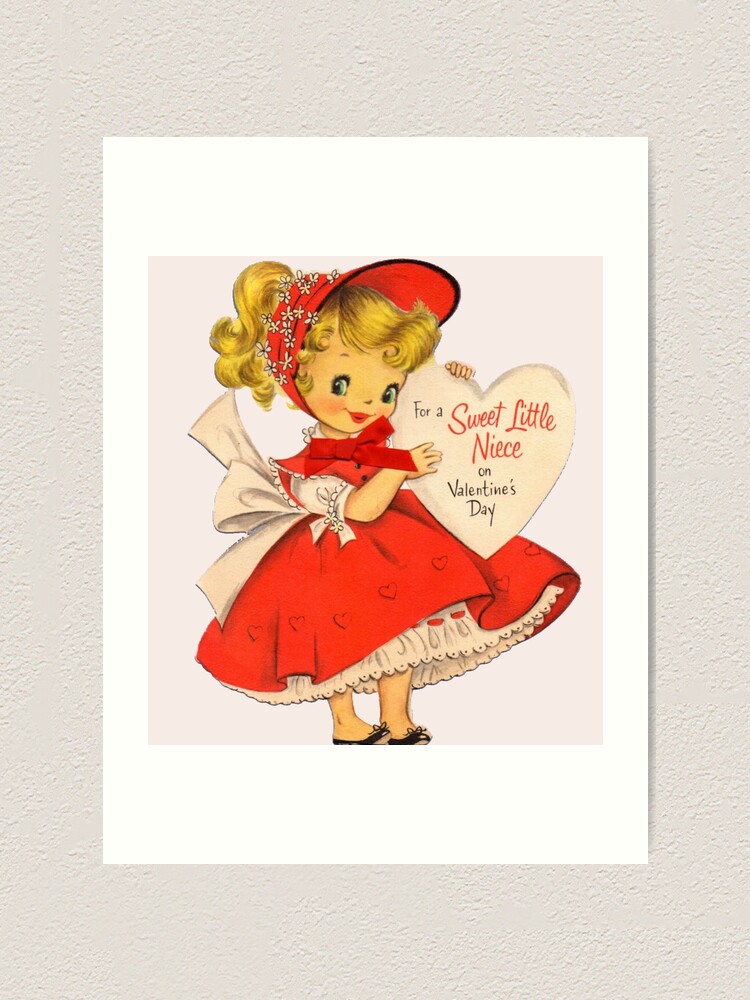This photograph captures a vintage-style Valentine's Day card set against a neutral background. At the center of the card is a charming illustration of a blonde-haired little girl with fair skin, dressed in an elaborate red outfit. She wears a large red bonnet adorned with flowers and a furly red dress featuring a prominent bow tied at the back, with white sleeves peeking out. The dress itself has a lacy frill underneath, and she completes her outfit with black shoes. The girl is holding a large pink heart with the inscription "For a sweet little niece on Valentine's Day" and is facing forward with a happy, smiling expression and blue eyes. The card evokes a nostalgic, vintage feel reminiscent of the 1920s to 1940s, though the card stock appears relatively new. The only text present is the message on the heart she holds, adding to the card's classic aesthetic.